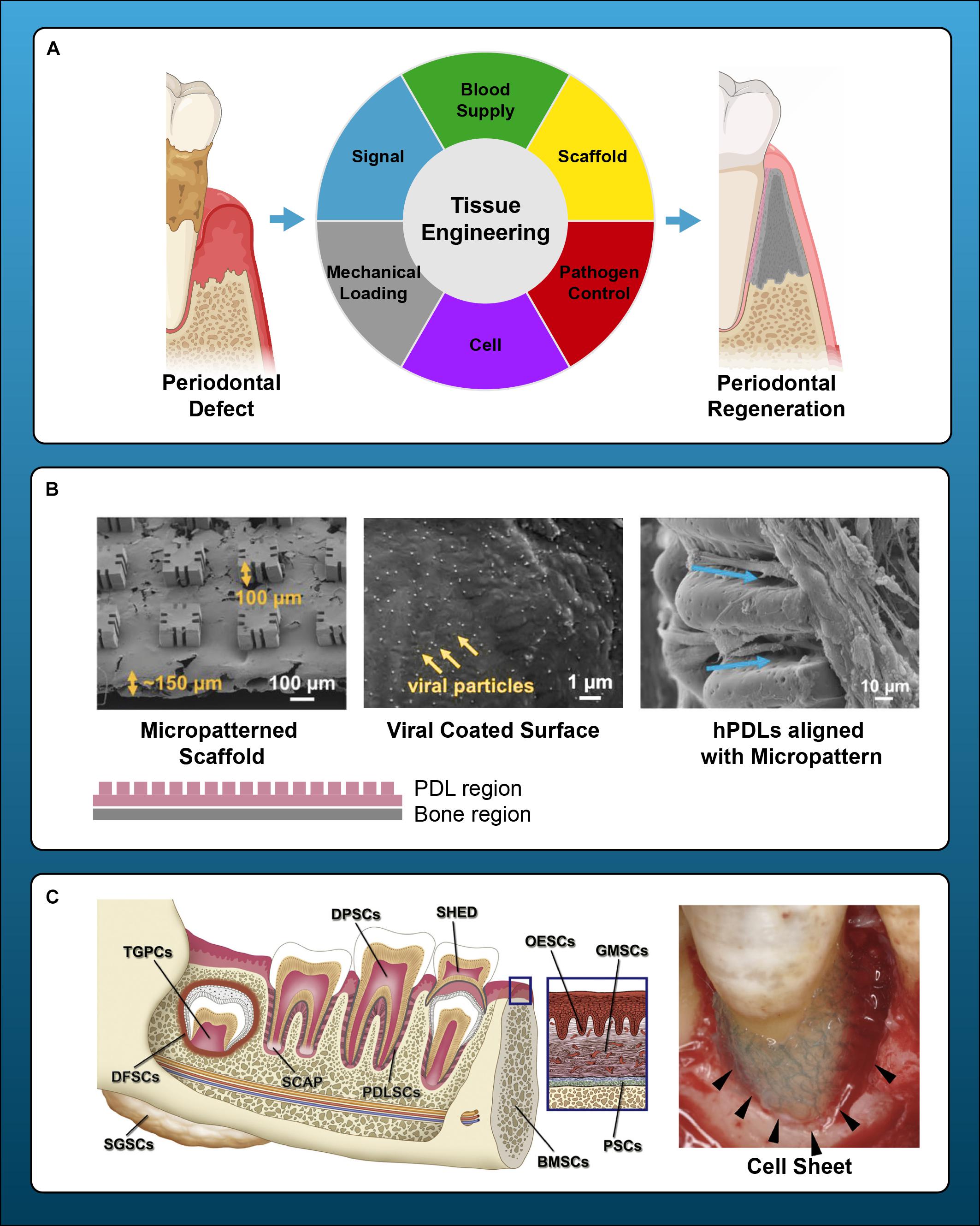This is a detailed scientific diagram displayed on a vertically aligned sheet with a gradient blue border, light at the top and darkening towards the bottom. The layout is divided into three horizontal sections, each representing different aspects of medical or dental science, set against a white background. 

The top section, marked 'A,' illustrates a color wheel centered around the concept of 'Tissue Engineering,' featuring segments in green, yellow, red, purple, gray, blue, and white with terms like 'blood supply,' 'scaffold,' and 'cell.' Flanking the color wheel are schematic images of teeth. The image on the left is labeled 'Periodontal Defect,' displaying a tooth with decay, while the image on the right is labeled 'Periodontal Regeneration,' showing repaired gum lining.

The middle section, labeled 'B,' contains a series of black and white microscopic images of dental cells. It includes three primary diagrams: 'Micropattern Scaffold,' 'Viral-Coated Surface,' and 'HPDL aligned with Micropattern,' each annotated with arrows and black text. This segment visually represents intricate cell structures and their alignment.

The bottom section, labeled 'C,' presents a cartoonish yet detailed anatomical drawing of a jaw, highlighting teeth and various cell pieces around it. The diagram meticulously labels each part of the tooth and gum structure, using black lines and text for clarity.

Overall, the image is a comprehensive educational tool detailing aspects of tissue engineering, microscopic dental structures, and anatomical illustrations of teeth and gums.